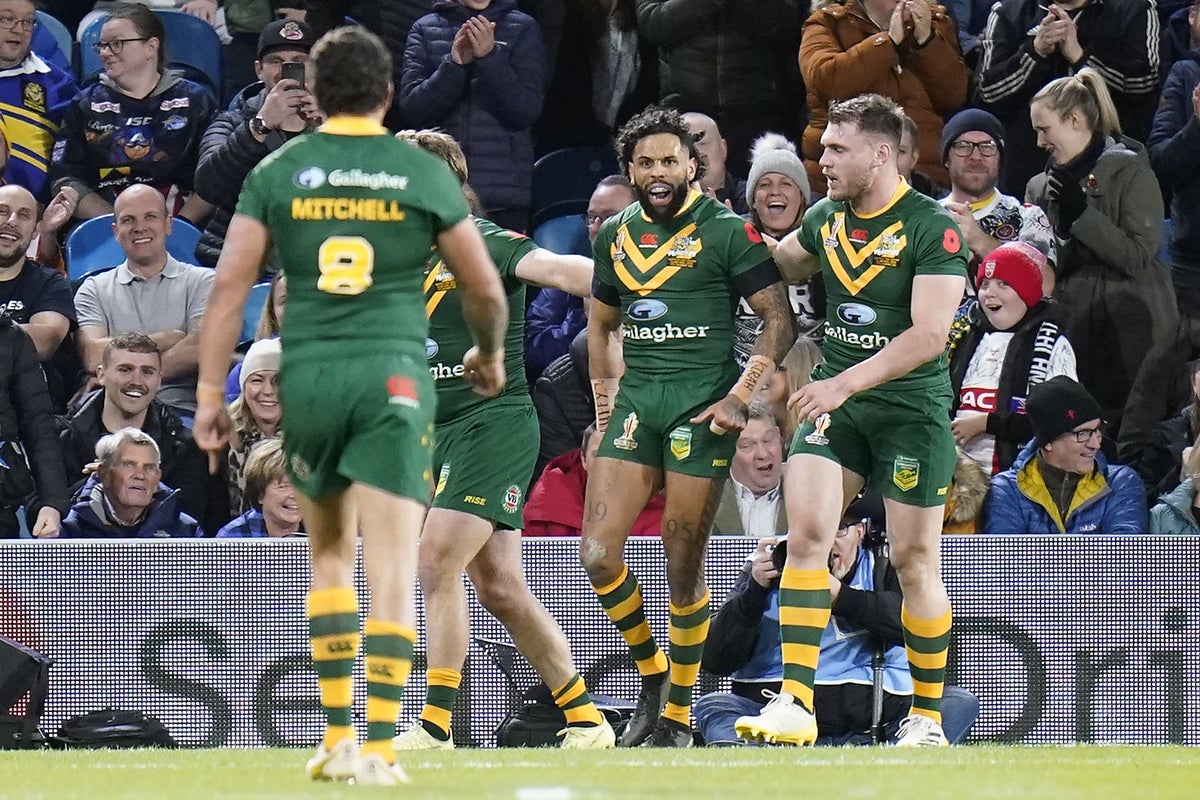The image captures an exhilarating moment at a rugby match, featuring four players wearing dark olive green jerseys with yellow stripes across the chest, paired with green shorts and yellow and green striped socks. The jerseys display a blue oval logo with a dark blue letter "G" and the word "Gallagher" underneath. At the center of the image is a black player with curly hair, energetically shouting in a victorious manner, facing directly towards the camera. He is flanked by two white teammates, one of whom is patting him on the back. The name "Mitchell" with the number eight is visible on one player's back. All players appear both exhausted and elated, sharing an intense moment of celebration. In the background, a lively crowd extends at least four rows deep, with spectators exhibiting a mix of joy and amazement. One fan is even capturing the scene with their cell phone, adding to the electric atmosphere of victory. The bottom of the image reveals a light green field and an LED advertising board, heightening the sense of a professional sporting event.